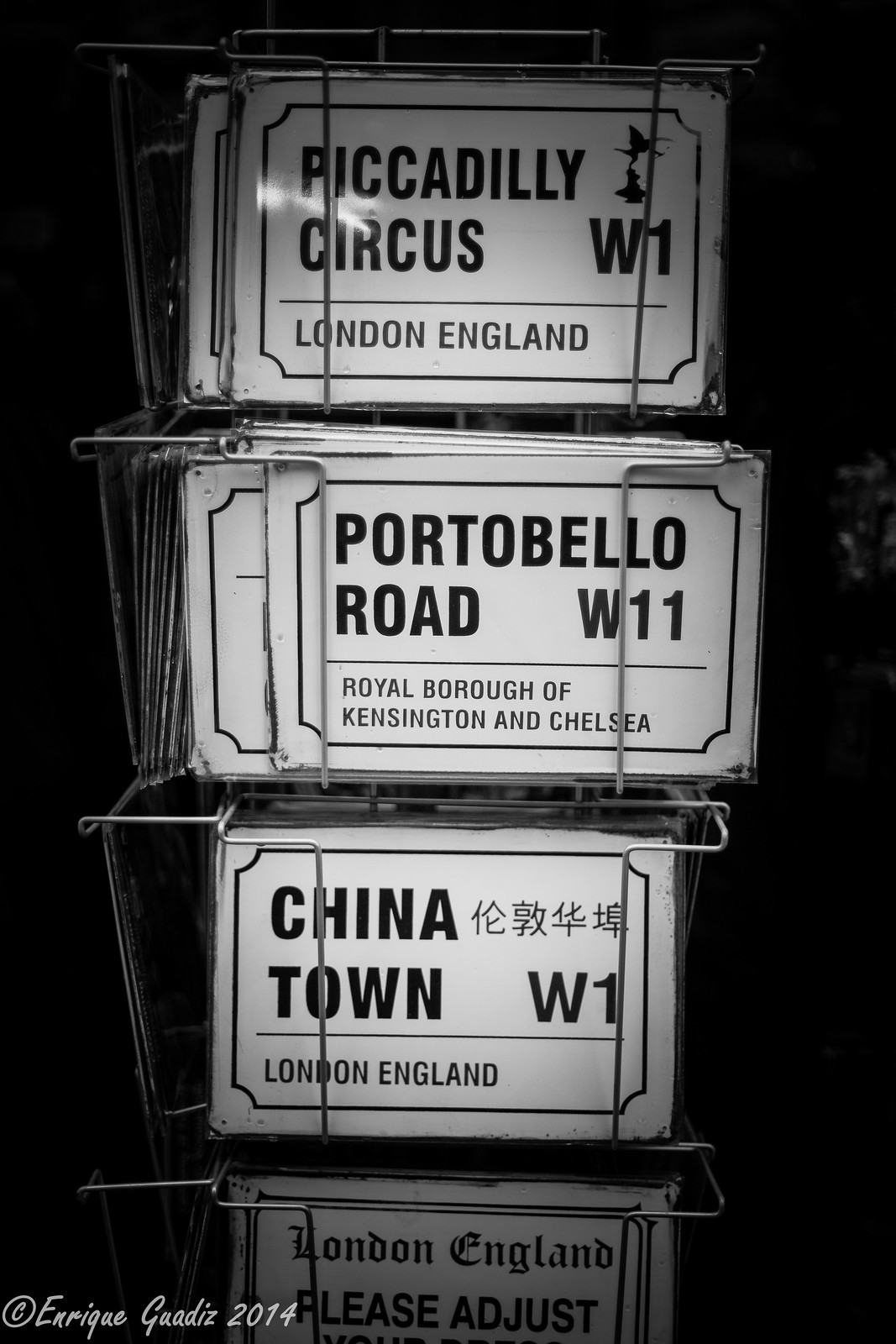This black-and-white photograph, taken by Enrique Gadez in 2014, captures a display of stacked road signs for sale, likely in a gift shop or souvenir area. Each stack is neatly organized on metal racks, with several identical signs in each vertical stack. The signs are characterized by a consistent design: black text on a white background with a thin black border. At the top of the display, the prominent sign reads "Piccadilly Circus, W1, London, England." Below it, another sign reads "Portobello Road, W11, Royal Borough of Kensington and Chelsea." The third sign in the stack showcases "Chinatown, W1, London, England," alongside some Chinese characters. The bottom sign is labeled "London, England, please adjust." The composition is illuminated in such a way that the signs are the focal point, standing out brightly against the darker, unlit background. The lower-left corner of the image bears the photographer's copyright mark, "Enrique Gadez, 2014," anchoring the timeframe of this evocative snapshot.